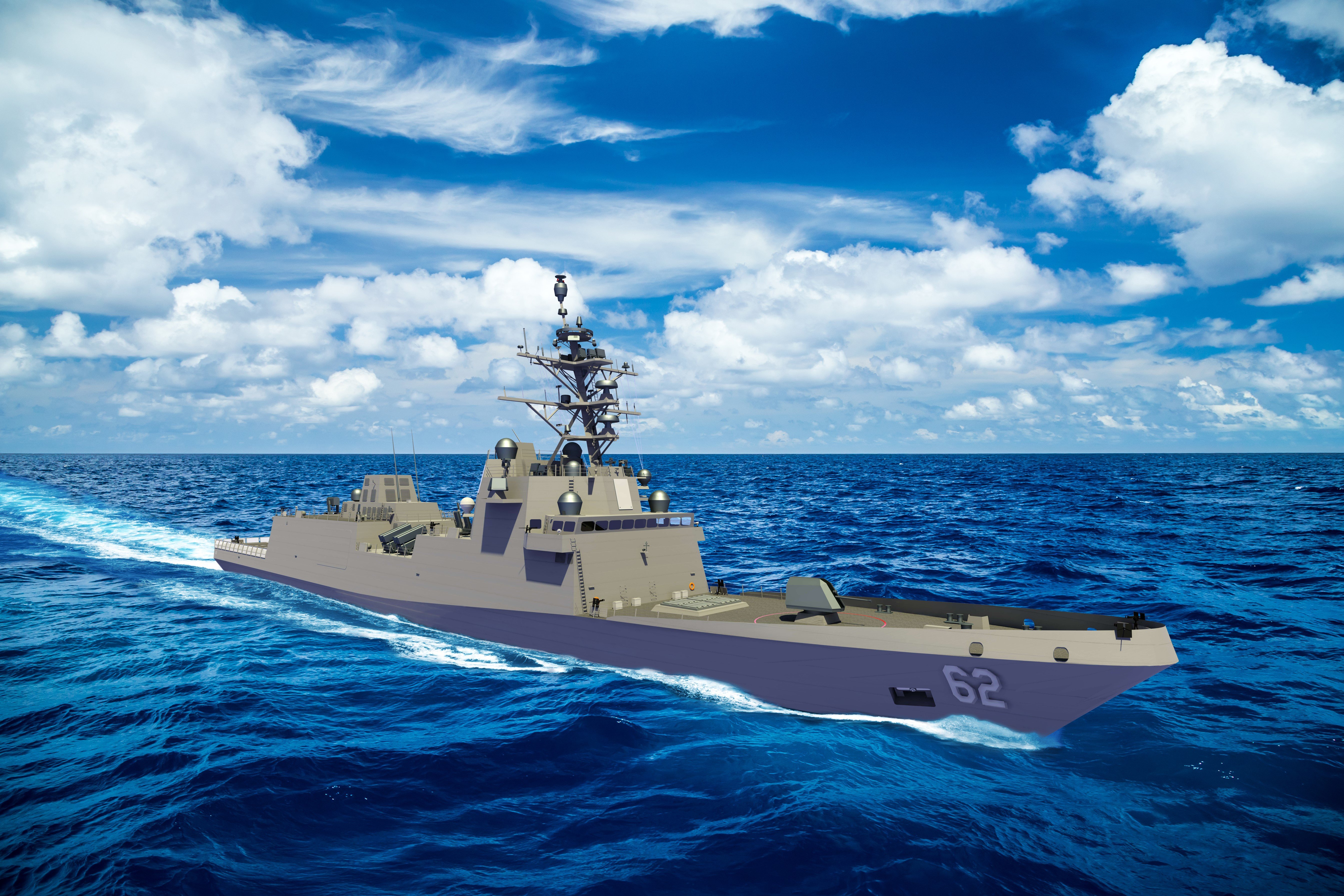The image depicts what appears to be a computer animation of a naval battleship, specifically marked with the number 62 in white paint on its front side. The ship is rendered in varying shades of gray, with a darker gray at the bottom and a lighter gray on top, indicative of a military vessel. It features a long forward deck that rises in the middle where a large lookout area or captain's command center is located, which is equipped with extensive radar and electronic equipment. Toward the rear, the ship descends back to a lower deck. On the sides, you can observe cannons and other weaponry, hinting at its battleship capabilities.

The ship is depicted cruising through a vibrant blue ocean, with the water's surface showing slight waves and a churning wake behind the vessel, illustrating its motion toward the lower right corner of the image. The sky above is bright blue with numerous clouds, suggesting a sunny day. Although the entire scene—including the ship, sea, and sky—appears vividly detailed, it possesses characteristics of digital creation, leading to speculation that it could be an element designed for a video game or other digital media. No crew members are visible on the ship, which also features a rear deck with additional antennas and equipment. The composition is in landscape orientation, with the open ocean dominating the lower half of the image and the expansive sky filling the upper half.